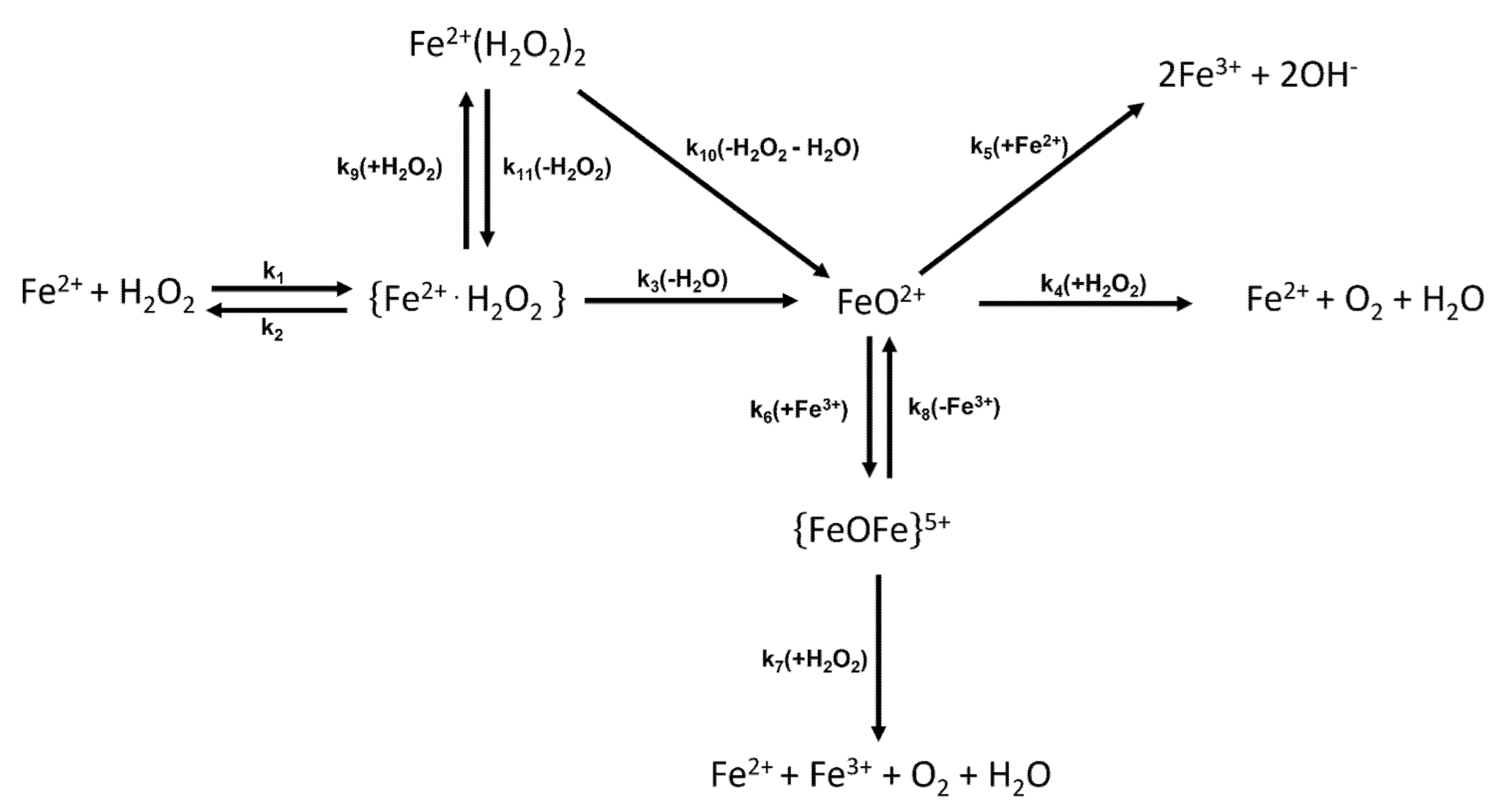The image is a complex chemical flow chart, likely designed for educational purposes within a laboratory or taken from an academic textbook. The chart features numerous abbreviations of chemical compounds and reactions, including prominent ones such as O2 (oxygen), H2O (water), and Fe2+ (iron ion). It visually represents the relationships and reactions between these substances, showcasing how different chemicals combine and transform into new compounds. The diagram is densely packed with arrows and plus signs, indicating multiple connections and interactions between the elements. There is no accompanying key, making it challenging to decipher what each abbreviation stands for without prior knowledge. The central figure, FeO2+, branches out to various reactions such as 2Fe3+ + 2OH- and Fe2+ + O2 + H2O, illustrating the intricate processes involved in these chemical equations. The chart is presented with black lettering on a white background, clearly mapping out the complex web of interactions and formulas.